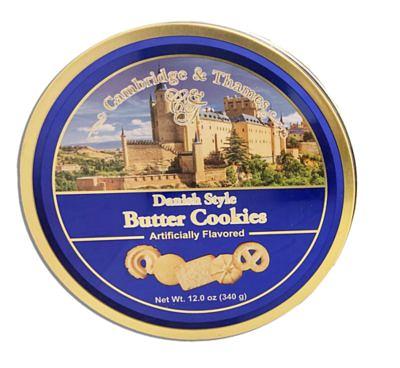The image displays a top cover of a circular cookie tin from Cambridge and Thames. The cover has a gold border with a predominantly royal blue background. At the top, "Cambridge and Thames" is elegantly inscribed in golden-yellow text, set against an image of an old European-style castle with large brick walls, blue rooftops, and surrounding hills and trees. Below the castle, the words "Danish Style Butter Cookies, Artificially Flavored" are written in matching golden-yellow text. The lower section showcases five distinct types of butter cookies, with shapes that include circular, rectangular, pretzel, and half-donut forms. The tin also marks the net weight as "12 ounces (340 grams)." The entire cover, featuring its intricate details and elegant design, sits against a white background.